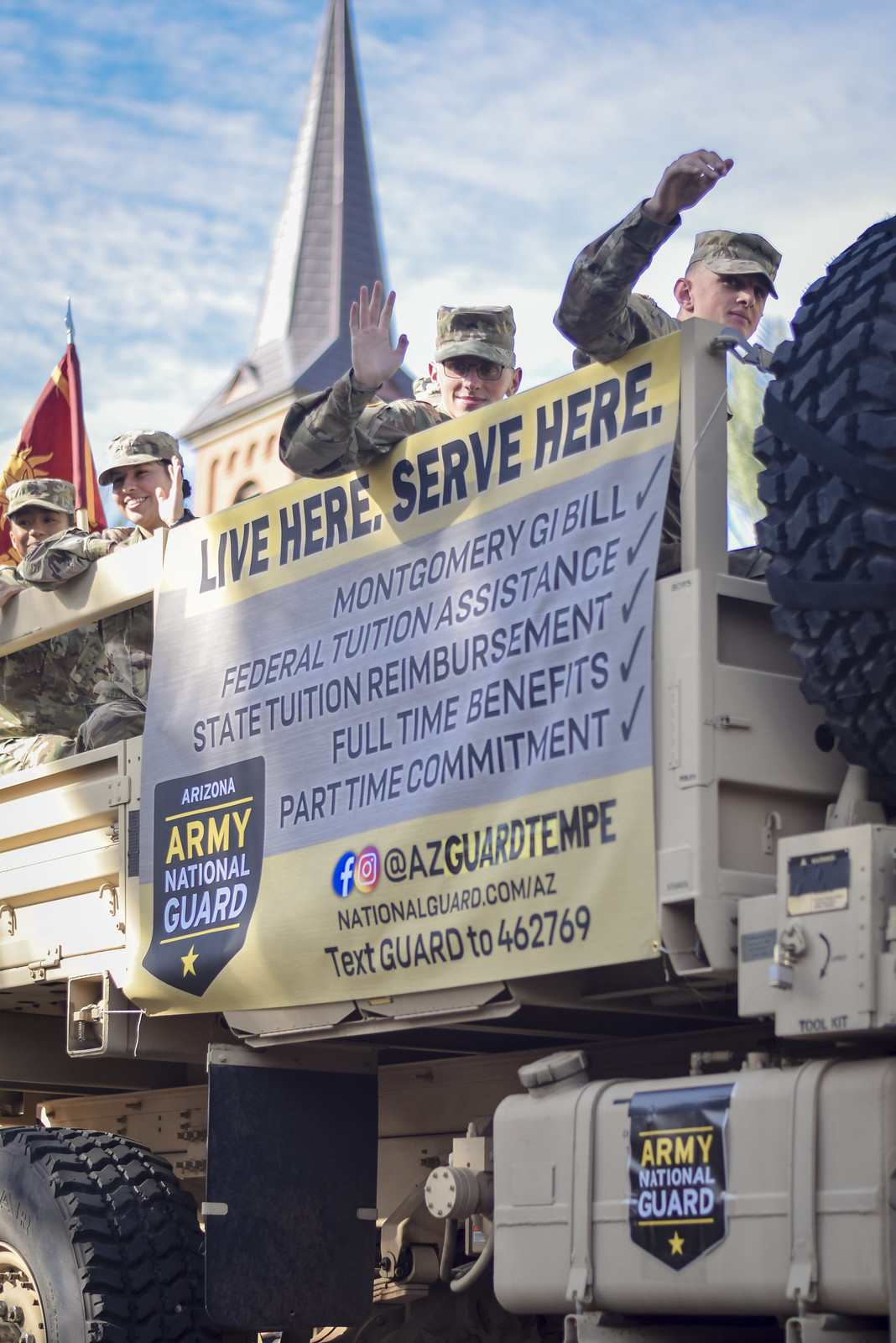In the photo, four service members from the Arizona Army National Guard, comprising two young women and two young men, are seen riding in the back of a beige, open-bed military transport vehicle. They are all waving towards an unseen entity, reminiscent of a parade scene. Prominently displayed along the side of the vehicle is a banner that reads, "Live Here, Serve Here," followed by five bullet points: "Montgomery GI Bill, Federal Tuition Assistance, State Tuition Reimbursement, Full-Time Benefits, Part-Time Commitment." The banner designates that they belong to the Arizona Army National Guard, with the statement “Arizona Army National Guard” on the left-hand bottom corner of the banner. Below the bullet points, social media handles for Facebook and Instagram are given as "@AZGuardTempe," along with more information available at "NationalGuard.com/AZ." An option to text "Guard" to 462769 is also provided. In the background, a church spire stands against a blue sky dotted with white clouds. The vehicle's exterior features additional emblems and signage, reinforcing the affiliation with the Army National Guard. Toward the bottom left, part of the tire is visible, and on the right, a gas tank appears to bear yet another "Army National Guard" label, adding to the detailed display of their identity and recruitment information.